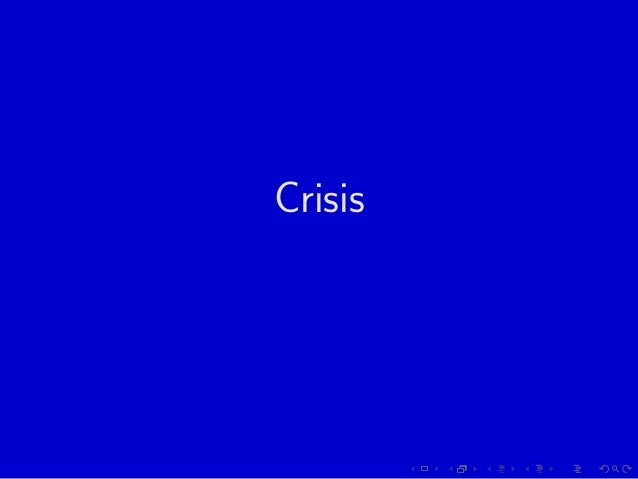The image features a vibrant, solid blue background that spans the entire square canvas. Centered both horizontally and vertically on this striking blue backdrop is the single word "Crisis," presented in white sans-serif text. The word "Crisis" begins with a capital 'C,' followed by the lowercase letters 'r-i-s-i-s.' Along the bottom right edge of the image, there are numerous small, light gray icons, including a rectangle, a pair of superimposed rectangles, dots, curved arrows pointing in opposite directions, and a magnifying glass. These subtle symbols are difficult to notice against the eye-catching blue background. Overall, the image appears to be a minimalistic graphic, possibly designed for a digital presentation or slideshow.